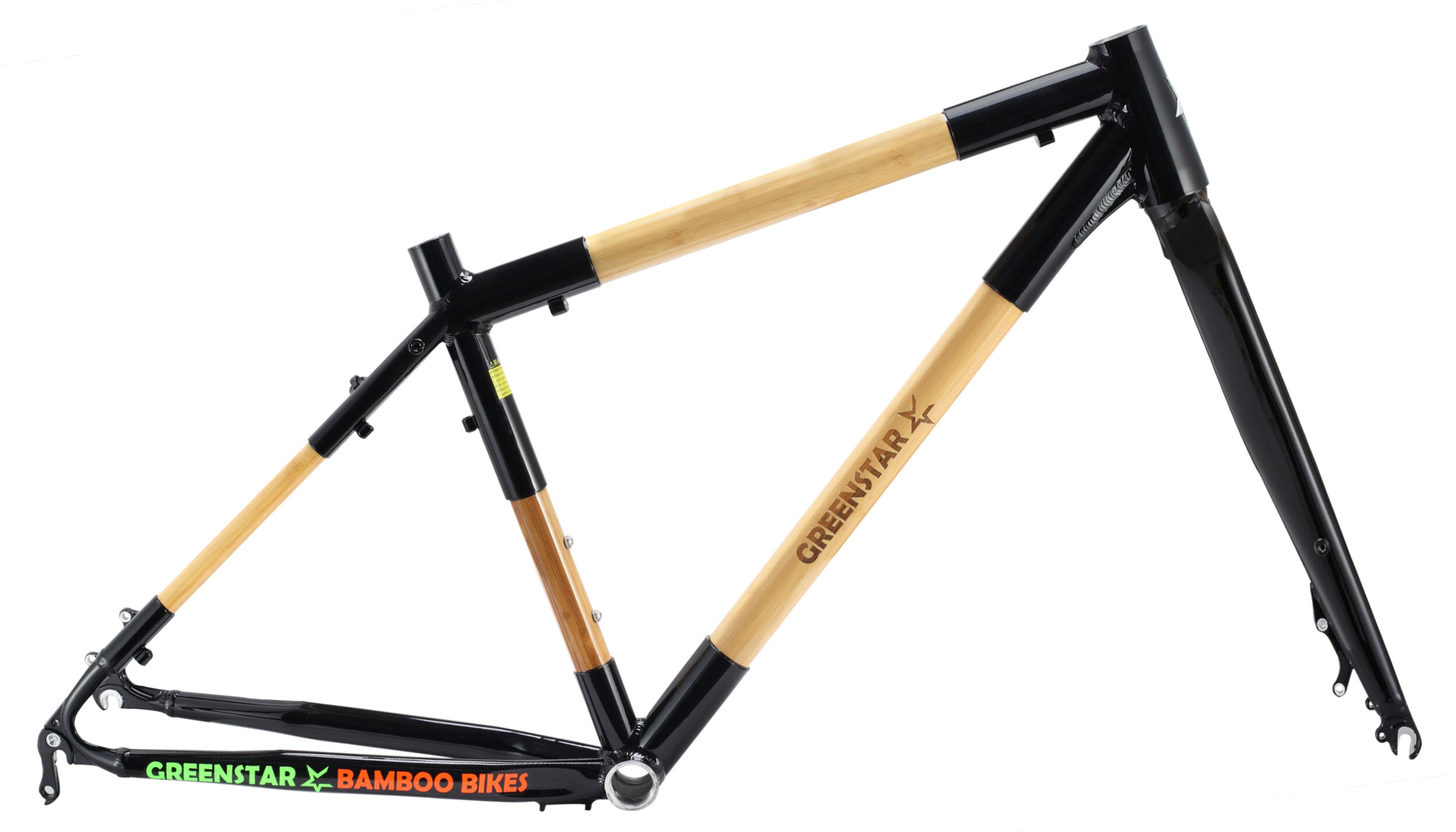The image showcases a detailed view of a bicycle frame placed against a solid white background. The frame features a combination of black metal on the edges and a beige, wood-like finish in the middle sections. The front of the frame is oriented to the right with the rear to the left. The frame forms two triangular shapes. The lower diagonal bar prominently displays the text "Green Star" in green letters, accompanied by a green star logo. Additionally, there is text in red letters that reads "Bamboo Bikes" near the rear of the frame, adjacent to a screw. The sophisticated design indicates a blend of wooden and metallic materials, capturing both aesthetic and functional elements. The high-quality image focuses on the intricate details including hooks and screws, emphasizing the craftsmanship of the frame.